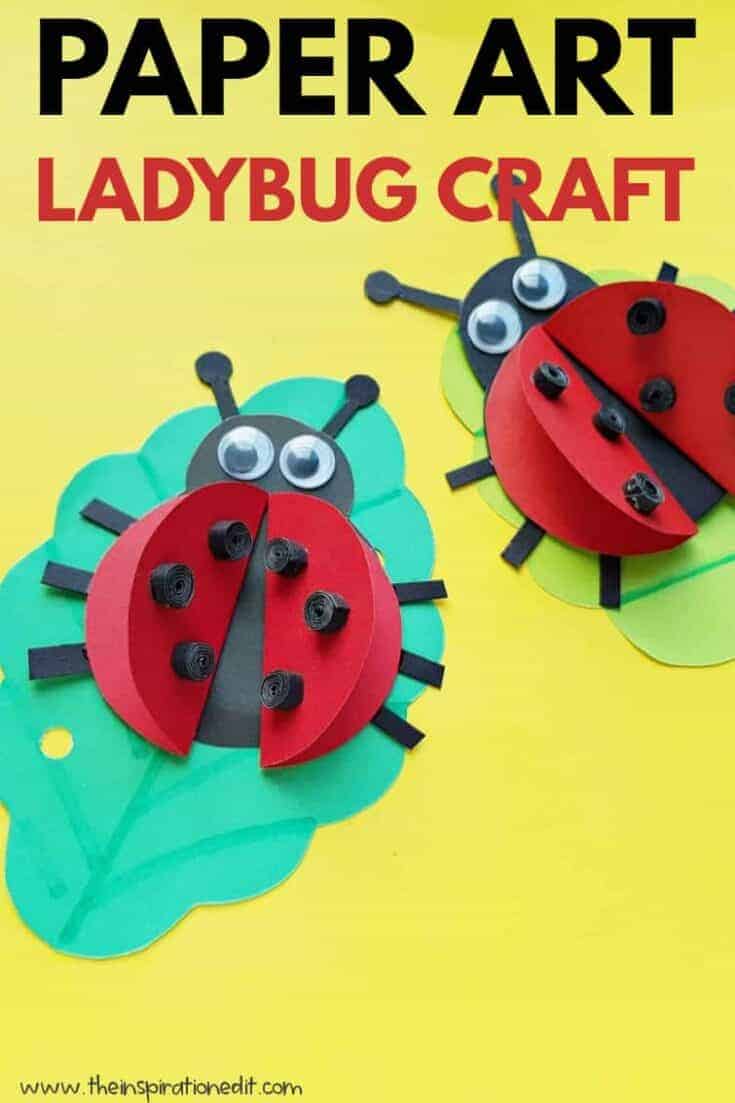The poster, promoting TheInspirationalEdit.com, showcases a vibrant arts and crafts project titled "Paper Art: Ladybug Craft" in bold black letters against a yellow background. Central to the design are two adorable paper-crafted ladybugs, each adorned with big eyes, intricate black spots, and delicate antennae and legs. The larger ladybug, in striking red and black, rests on a pale blue, meticulously cut-out leaf, while the smaller ladybug, similarly colored, perches on a neon green folded leaf. The poster exudes a playful and educational vibe, ideal for sparking creativity in kids. The website address is neatly positioned in the bottom left corner, tying everything together in this detailed and visually appealing advertisement.